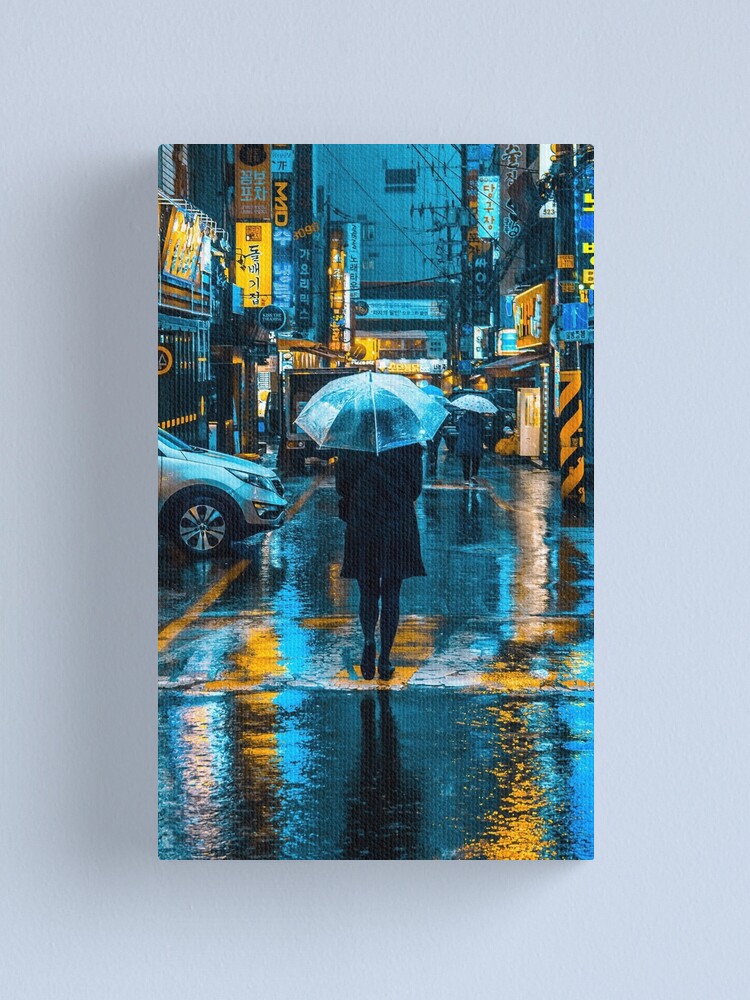In the dimly lit, rainy night of an Asian city street, a person is captured from behind, walking with a large clear umbrella shielding them from the rain. They are dressed in a black overcoat, black tights, and black shoes. The wet pavement reflects the city’s neon lights, casting a bright blue and yellow glow. The street is bustling with activity; ahead of the person, other pedestrians, also clad in dark clothes and carrying umbrellas, navigate the rainy roadway, highlighted by numerous store signs bearing Chinese or Japanese characters. To the left, a car’s hood protrudes into the street, adding to the urban scenery highlighted by power poles and the myriad of illuminated signs. The photograph, possibly twice as tall as it is wide, evokes a scene reminiscent of cities like Tokyo or a vibrant Chinatown, portraying the ambiance of an inner city drenched in rain.